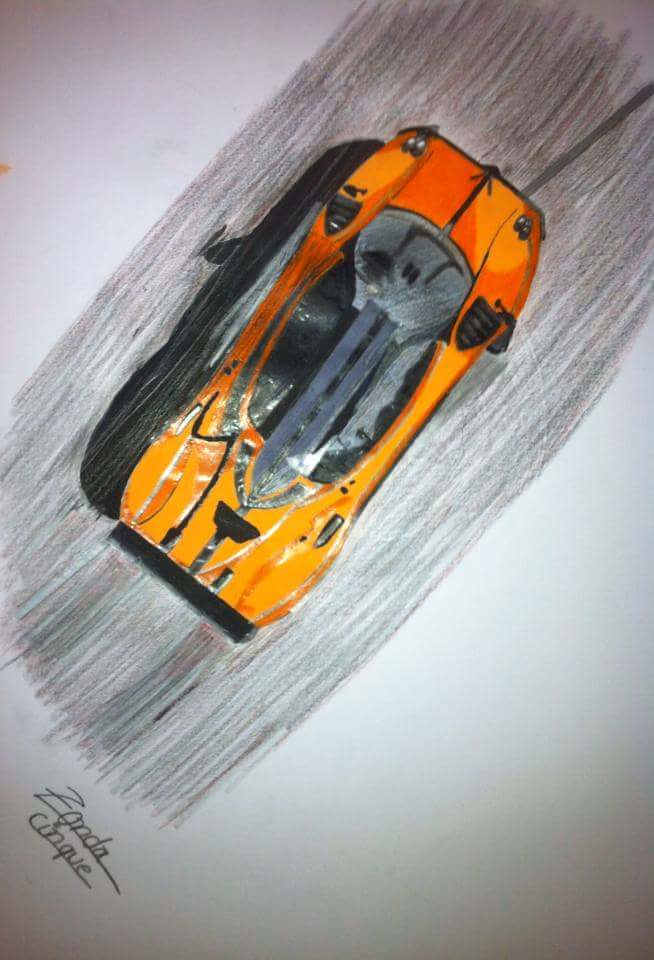An overhead pencil drawing meticulously illustrates an orange sports car, reminiscent of a Ferrari with its low-sitting, aerodynamic cabin and sleek design. The scene includes a shaded road, giving context to the car's position, and the vehicle dynamically casts a shadow, suggesting it is bathed in daylight. The artwork, signed "Zonda Cinque," captures the essence of a high-torque, high-horsepower race car without aligning fully with the traditional NASCAR style.